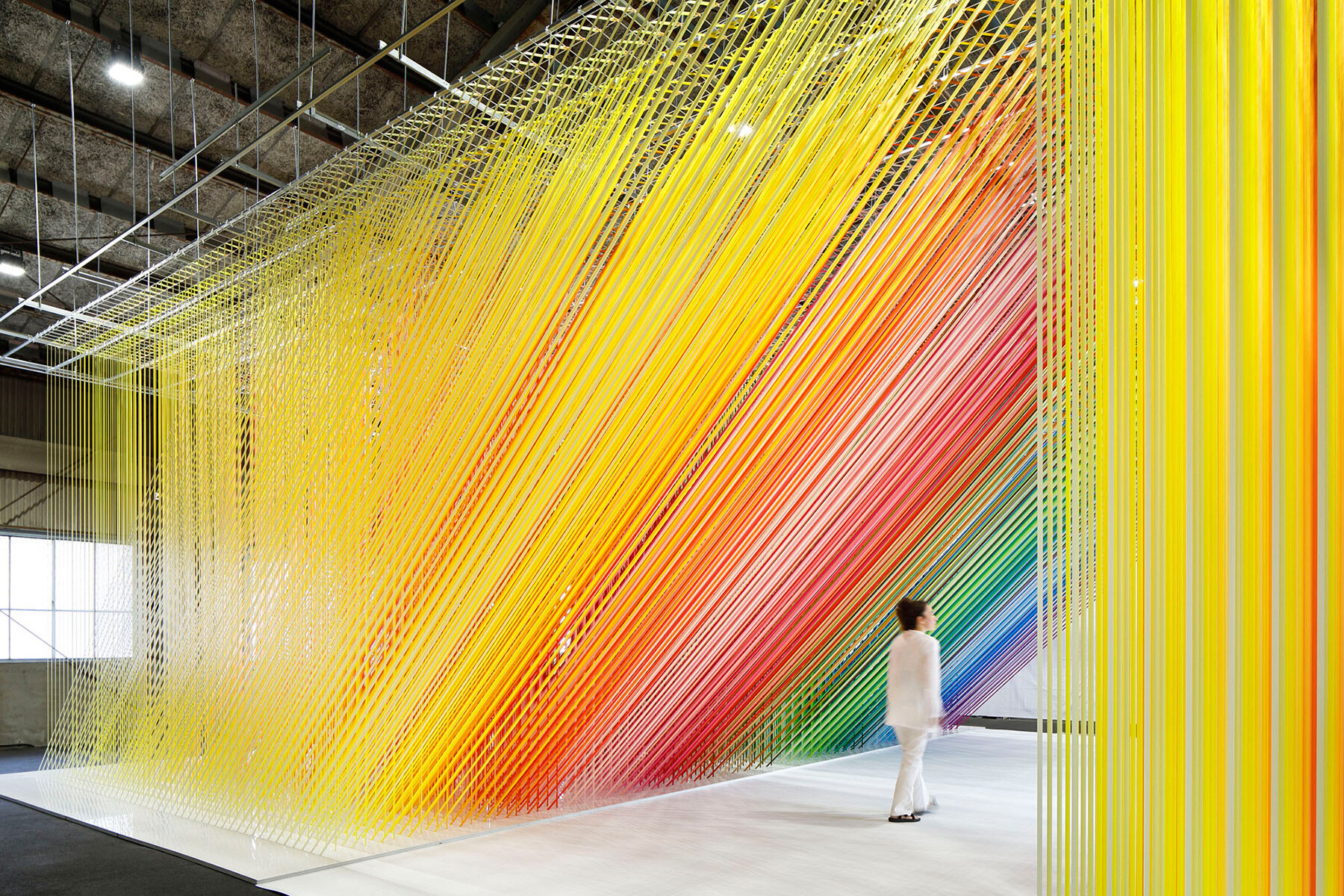The photograph depicts a vibrant and colorful installation inside a tall building, possibly a stage or a warehouse, characterized by its striking rainbow-hued decor. Various thin strands in vivid colors -- predominantly yellow on the periphery, transitioning through orange, red, green, blue, and purple as they converge diagonally towards the center -- hang down from metal rafters and poles attached to the ceiling. These colorful strands create a mesmerizing triangular archway that frames the scene.

At the center of this visually arresting display, a woman with dark hair styled in a bun, dressed in a striking white suit and black shoes, walks along the white floor. She moves beneath the cascading array of colorful strands, which impart a dynamic and artistic ambiance to the photograph. The diagonal and vertical arrangement of the multi-colored strings against the industrial backdrop of the building creates a captivating and immersive visual experience.